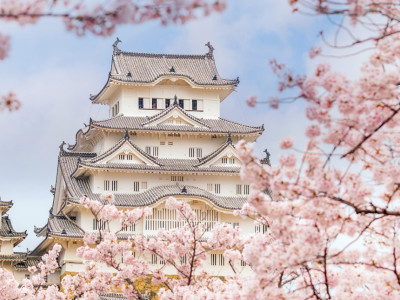This detailed image depicts a beautifully ornate multi-story Japanese pagoda, likely a temple, surrounded by lush cherry blossoms in full bloom. The tall white pagoda, which appears to have at least four or five stories, is characterized by its pointed, light gray roofs that curve elegantly outward, complete with traditional fish decorations on the corners. The structure features numerous slatted black-line windows on each level, enhancing its intricate design. Framing the image are vibrant pink and purple cherry blossoms that add a burst of color to the scene, almost as if you're peeking through a natural floral frame. The sky above is a mix of blue and white, with clouds dotting the serene backdrop. The detailed setting captures the pagoda from a zoomed-out perspective, allowing for an appreciation of the harmonious balance between the ornate architecture and the surrounding natural beauty.